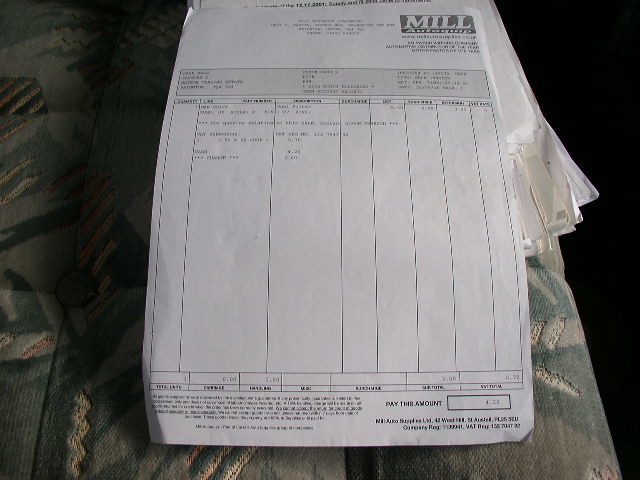This image depicts a blurry, low-resolution photo of a square-shaped sheet of paper positioned prominently in the center. The paper in the foreground is white with black print, though its contents are difficult to discern due to the image's poor quality. The top right corner of the paper features the text "Mills," followed by the word "Antique" beneath it. Below these headings is a block of black text that remains largely illegible. In the background, additional sheets of paper are visible, though they, too, suffer from the overall fuzziness and pixelation of the image.